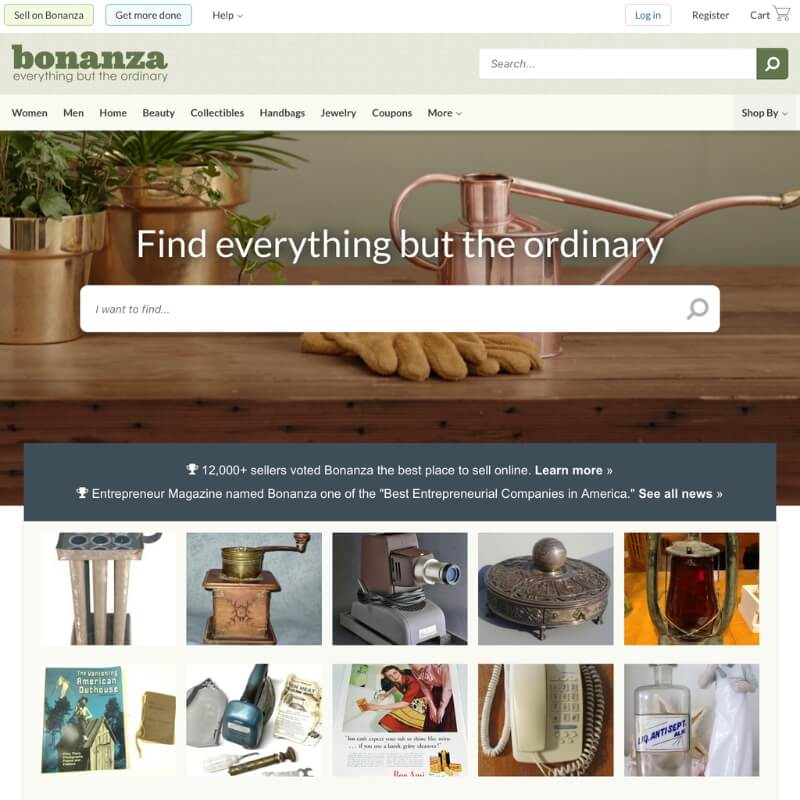This is a screenshot of a website, showcasing the user interface and navigation elements in intricate detail. 

At the very top, there is a white navigation bar. On the left side, a beige button labeled "Sell on Bonanza" appears in black font. Next to it, a gray button reads "Get More Done." Following that is a drop-down menu labeled "Help." On the right side of the bar, there is a "Login" button in blue font, followed by "Register," and a cart icon indicating the shopping cart feature.

Below the white bar, a beige rectangular section features the website's slogan in brown font: "Bonanza: Everything but the Ordinary." To the right of this slogan is a search field for user queries.

Beneath this section, there is a lighter beige bar containing category labels in brown font: "Women," "Men," "Home," "Beauty," "Collectibles," "Handbags," "Jewelry," "Coupons," and "More."

The main content area of the screenshot shows a photograph of a rustic, rough-looking wooden counter. On the counter, there are two potted plants, a watering can, and a pair of work gloves. Overlaying this image is a text in white font that reads "Find everything but the ordinary," followed by another search field labeled “I want to find…”

At the bottom of the image, there is a gray rectangular section, completing the user interface elements visible in the screenshot.